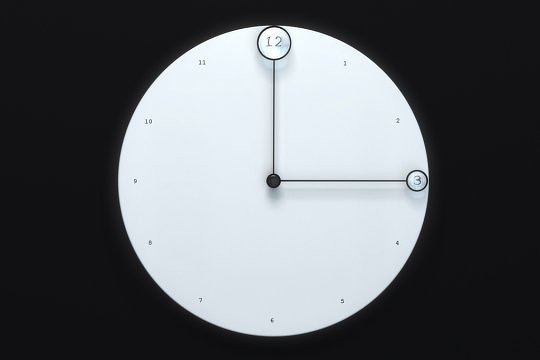The image showcases a minimalistic, computer-generated modern clock with a clean white circular clock face set against a contrasting black background for emphasis. The clock features Roman numerals distributed around its circumference, but no additional markings. Notably, the clock lacks traditional hands and instead employs two long, slim rods ending in circular, magnifying glass-like structures. The larger circular magnifier at the end of the hour hand enlarges the Roman numeral XII (12), and the smaller circular magnifier at the end of the minute hand enlarges the Roman numeral III (3), indicating the time as a quarter past twelve. The image's distinct details, such as the magnifying glass effect at the ends of the hands and the absence of conventional tick marks or hashes, emphasize its modern, minimalistic design.